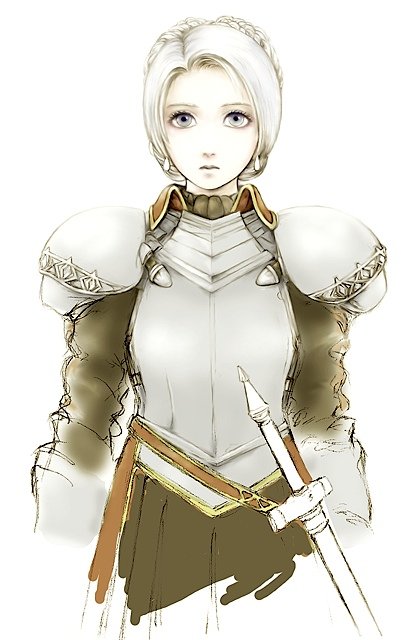This detailed anime-style illustration portrays a young woman in knight armor, characterized by her striking blonde hair styled into a braid and her large, expressive blue eyes. Her face appears calm and focused, with small, pursed lips. The armor is intricately designed, featuring prominently large shoulder pads etched with diamond shapes and a fitted metal chest plate. She wears a brown and brownish-green frock-like vest beneath the armor, along with a dark brown skirt—though the illustration cuts off at her thighs, giving it an incomplete, sketch-like appearance. A long sword, emblematic of her readiness for battle, hangs from a brown belt at her hip. Subtle details, such as her earrings, add to the depth of her character, conveying a warrior's calm amidst the anticipation of combat.